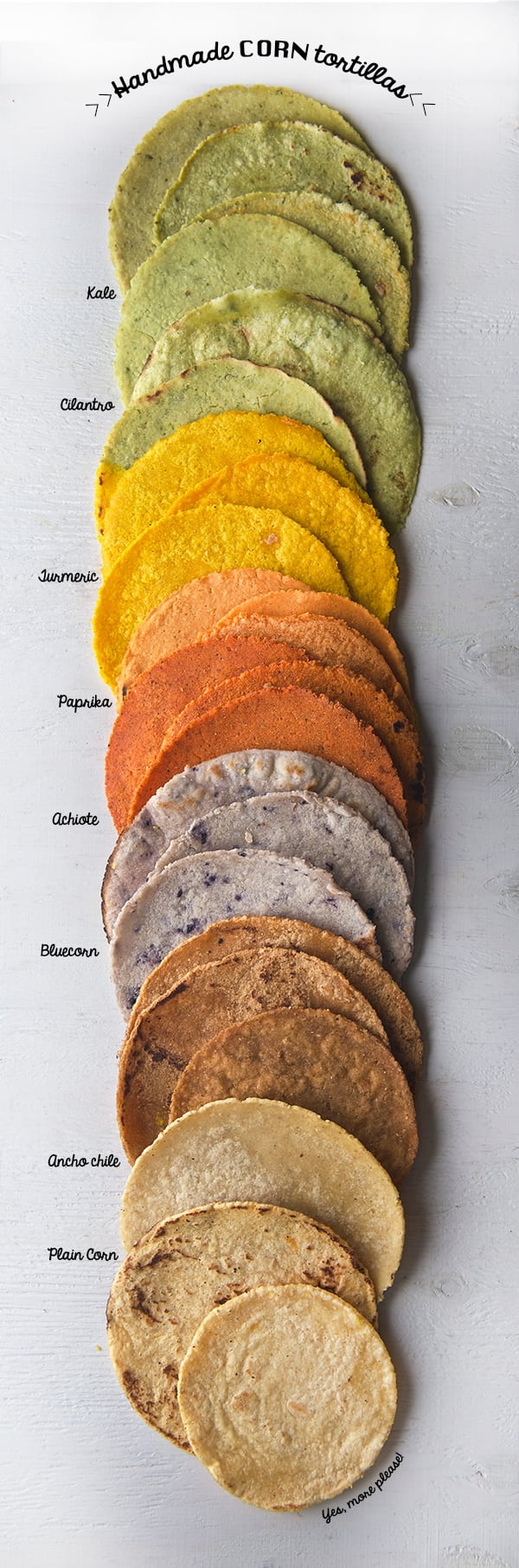The photograph is a vertical, high-quality image titled "Handmade Corn Tortillas," with curved black text at the top. It showcases a row of tortillas laid out on what appears to be linen paper, which features printed words along the left side, although some are too small to read clearly. The tortillas are arranged in a gradient of colors, from green at the top to plain corn at the bottom, highlighting the variety of flavors. The topmost tortillas are green, made with kale and cilantro, followed by yellow tortillas made with turmeric, orange tortillas flavored with paprika, and a purple or blueberry-hued tortilla. The photograph effectively illustrates the array of tortilla flavors transitioning smoothly from one color to another, with each one distinctly shaped and edged.